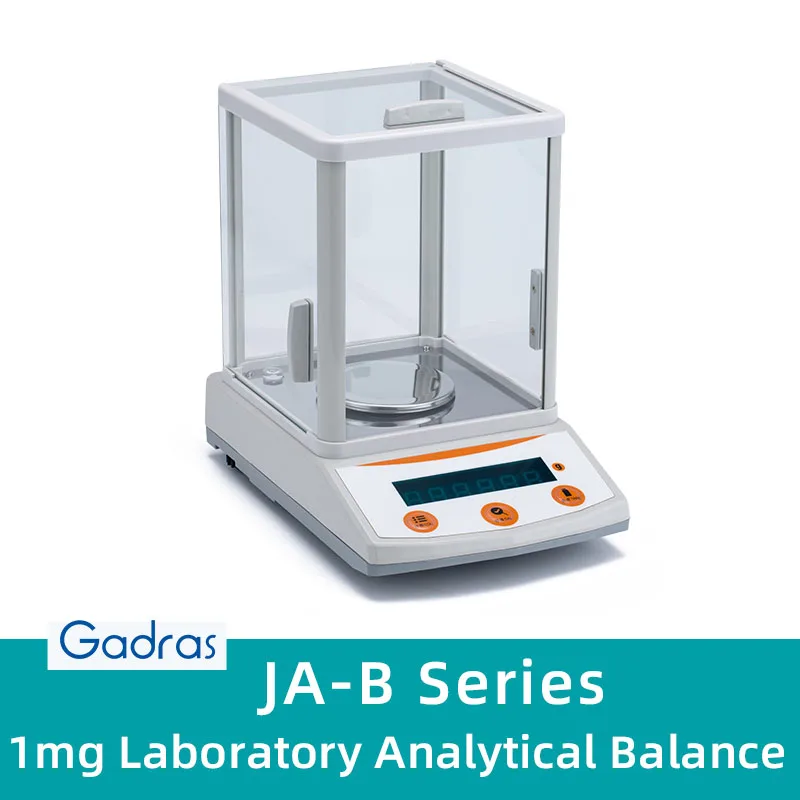The image depicts a laboratory analytical balance used for scientific experiments. Set against a flat white background, the contemporary-designed device features a gray base reminiscent of a grocery store fruit scale. Front and center are three round, orange buttons set against a white backdrop, accompanied by a digital panel for readouts. The weighing platform is enclosed in a transparent, glass box with small doors on all four sides, providing easy access to the circular silver pedestal inside. Reinforced columns support the glass case, adding to its modern aesthetic. At the base of the image, the text "GADRAS" appears in blue, while a teal rectangle houses the label "JA-B Series, 1 mg Laboratory Analytical Balance" in white, highlighting its precise measuring capabilities.